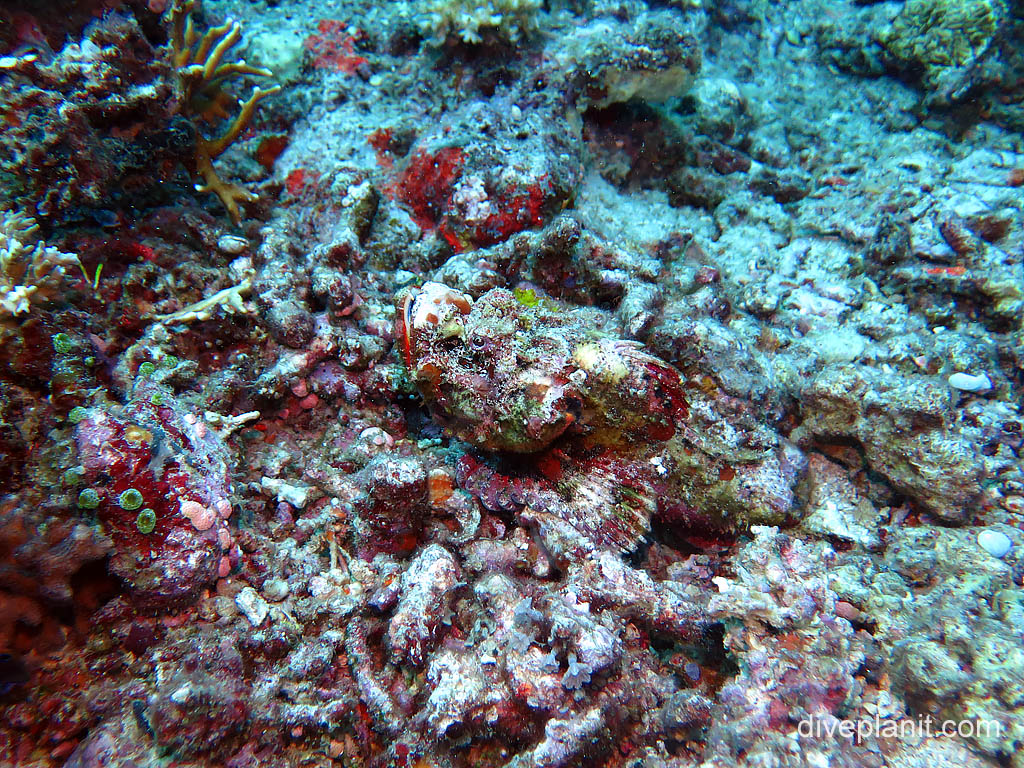The image depicts a detailed and colorful section of the seafloor, illuminated by natural daylight filtering through the water. The rocky terrain, predominantly gray, is interspersed with vibrant specks of red and green. The bottom portion of the image reveals rocks imbued with a light purple hue mixed with red, transitioning to a light blue hue towards the top. Notably, in the center, there is a large, multicolored rock that stands out amidst the surrounding textures.

In the top left and top sections, clusters of green plants are visible, with those in the top left resembling thick asparagus spears, adding a touch of lushness to the rocky landscape. On the left side, additional water plants that are white and spear-like can be seen, contrasting against the dark gray rocks behind them.

The bottom left corner showcases barnacles in varied colors of green, pink, and white, alongside small pieces of shell embedded in the jagged rock surface, and patches of reddish algae that taper off into the more prominent blue hues. The bottom right corner of the image features a watermark reading "diveplanit.com," where 'planit' is uniquely spelled.